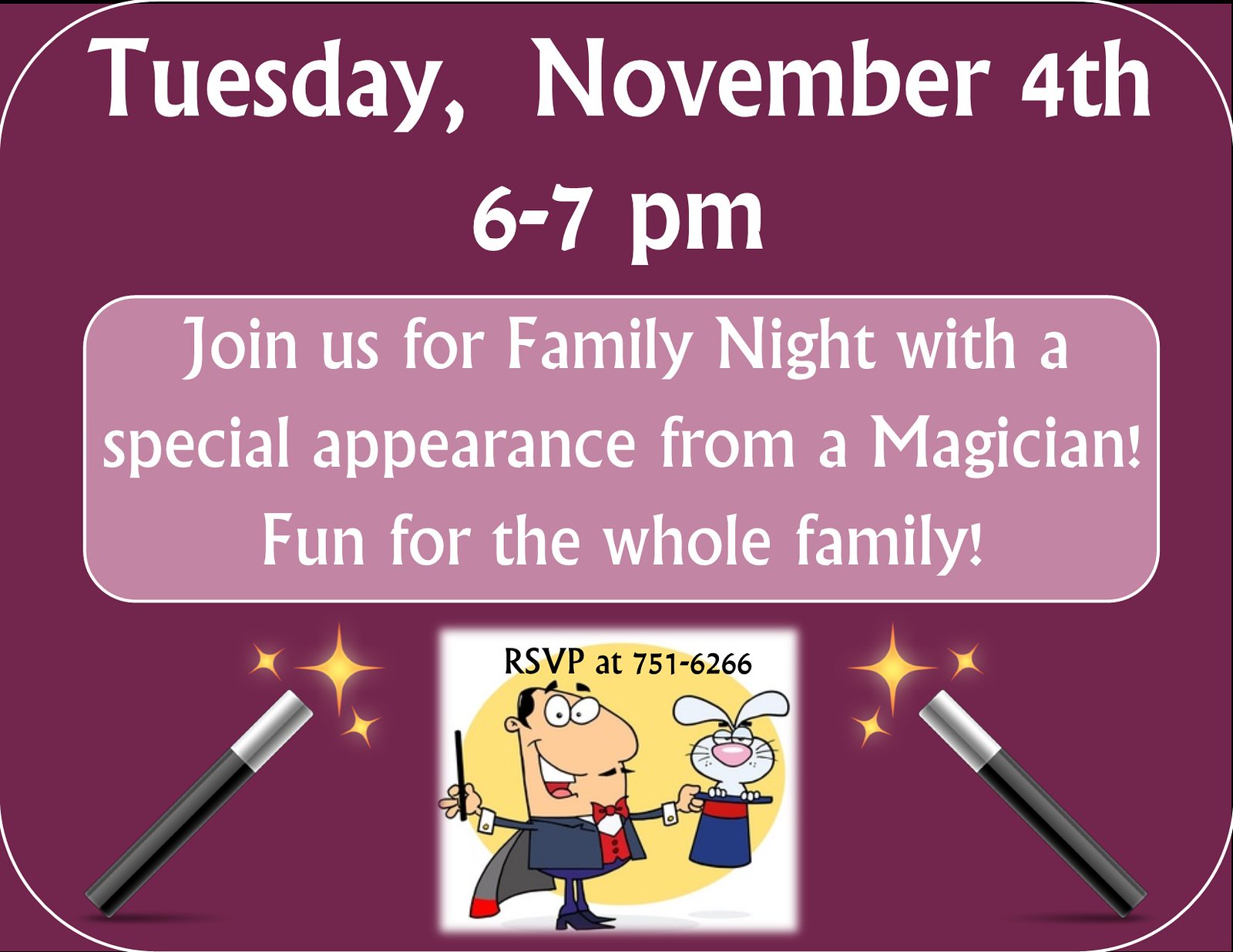The image features a vibrant purple background announcing an event. At the top, bold white text reads, "Tuesday, November 4th, 6 to 7 p.m." Below this, a lighter pink rectangular box with a white outline invites viewers to "Join us for Family Night," emphasizing "Family Night" with capital letters. It continues with, "with a special appearance from magician The Amy," all in white text, ending with an exclamation mark. Another line declares, "Fun for the whole family!" Also with an exclamation mark. In the bottom corners, there are decorative elements: a magician's wand with a black handle and a white tip, surrounded by stars. In the bottom center, an illustration shows a magician holding a hat from which a bunny with an impressed expression is emerging. Above the magician, it states, "RSVP at 751-6266."